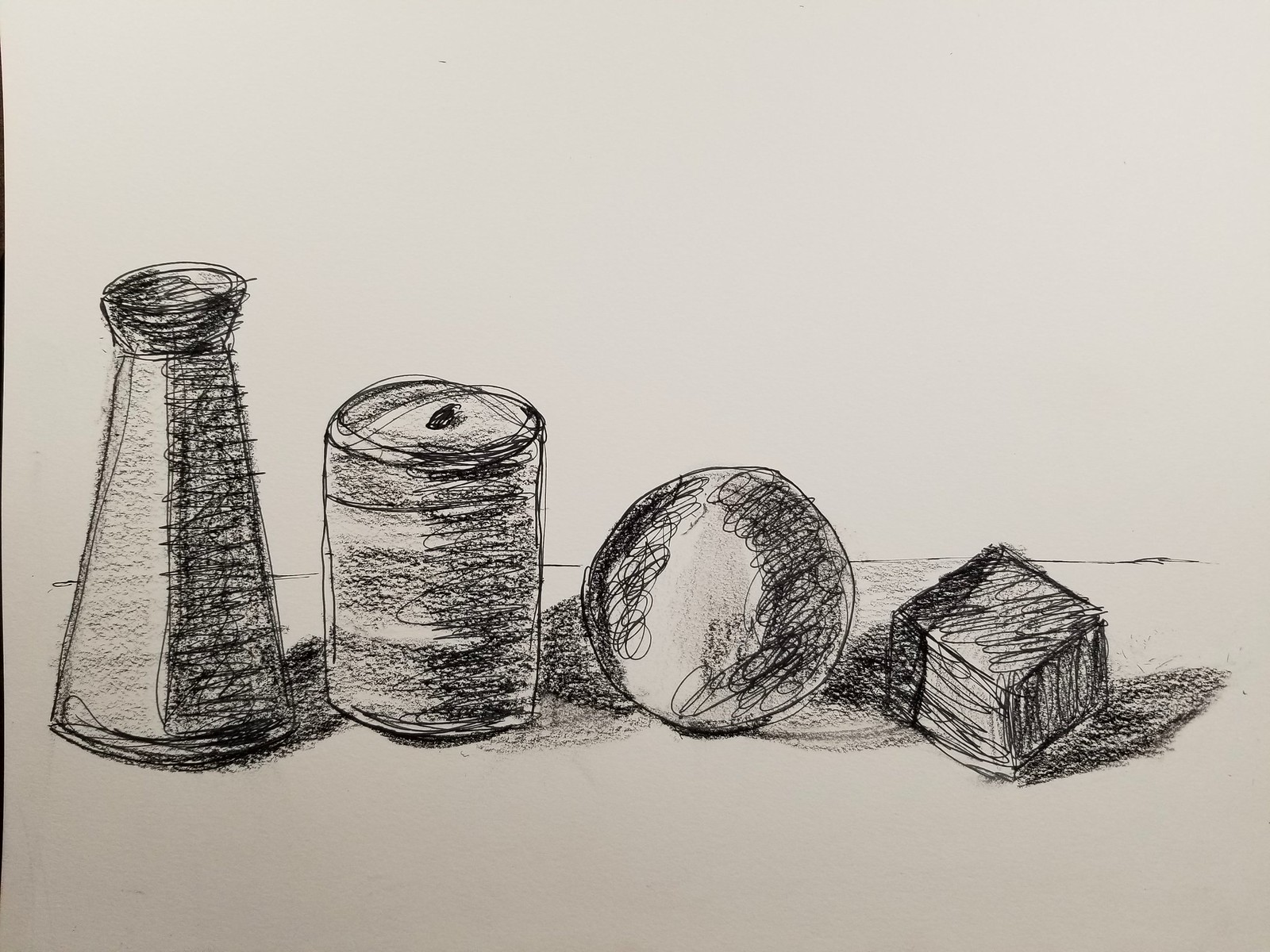This black and white sketch, drawn with pencil or charcoal, features a series of objects arranged on a table. The left side showcases a tall, cylindrical object resembling a salt shaker or perhaps a can with an opening at the top. Moving toward the middle, to its right, there is a rectangular jar with a lid. Further to the right, a sphere is placed next to a small cube. Each object is accompanied by shadows, giving them depth and dimension. The drawing is crudely rendered in black pen or pencil, with the right side more heavily shaded implying an irregular light source. This simple yet precise artwork, potentially a class assignment, uses basic geometric shapes and shadows to emphasize form and structure.